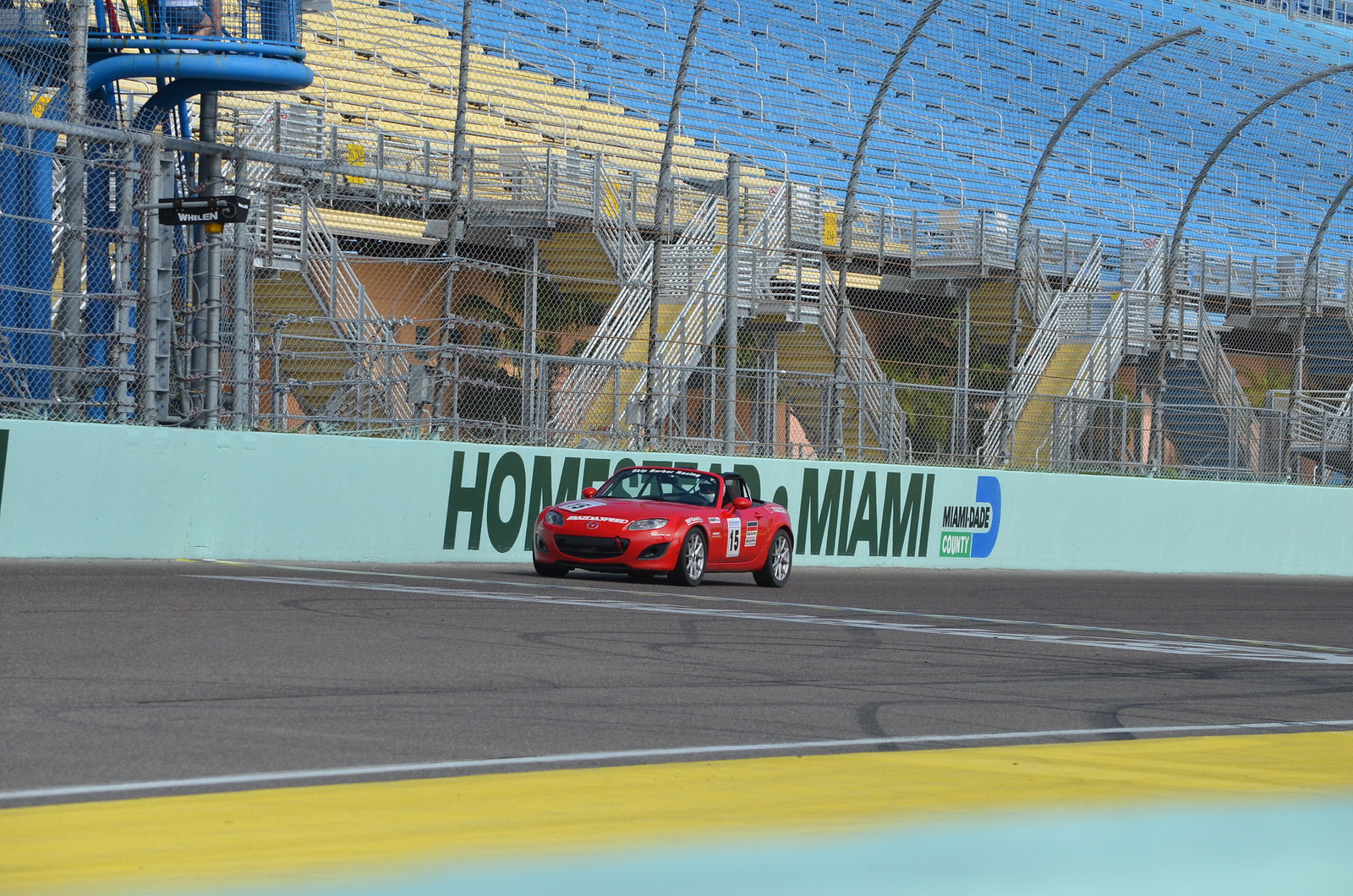The photograph depicts a large, outdoor racetrack viewed from the inner part of the track, facing towards the empty stands. These stands are divided into blue and yellow sections and feature three sets of stairs for access. The scene is likely from a practice session, as there are no spectators present. A small red convertible, resembling a Mazda Miata with the number 15 and various sponsorship logos, is positioned on the track near a white line and some visible skid marks. The car is slightly angled to the left, facing towards the viewer. In the background, a protective boundary surrounds the track, painted in a light mint green color. This boundary prominently displays the text "Homestead Miami" in large, dark green letters, though the car partially obscures the word "Homestead." Above the boundary, poles curve inward, supporting a net that stretches between the boundary and the stands. This comprehensive setup highlights the racetrack’s scale and readiness, even in the absence of a crowd.